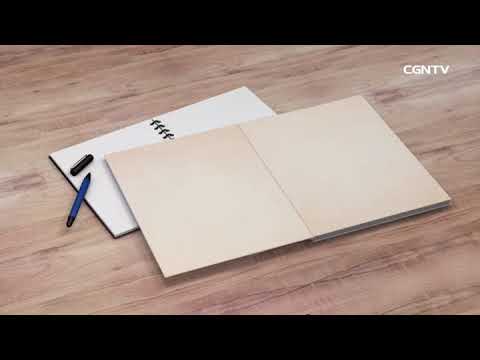This photograph captures a detailed scene of a wooden tabletop with a diagonal grain pattern in lighter wood and darker striations, adorned with two open books and a pen. In the top right corner, white text reads "CGNTV." Centrally, there is a larger book with its cover open revealing blank, tan-colored pages. Beneath this book lies a smaller spiral notebook featuring a black cover and a black wire spiral along its middle, opened to blank, crisp white pages. To the left, at a diagonal, rests a blue pen with its black cap removed and placed beside it, adding a touch of contrast to the earthly tones of the composition.